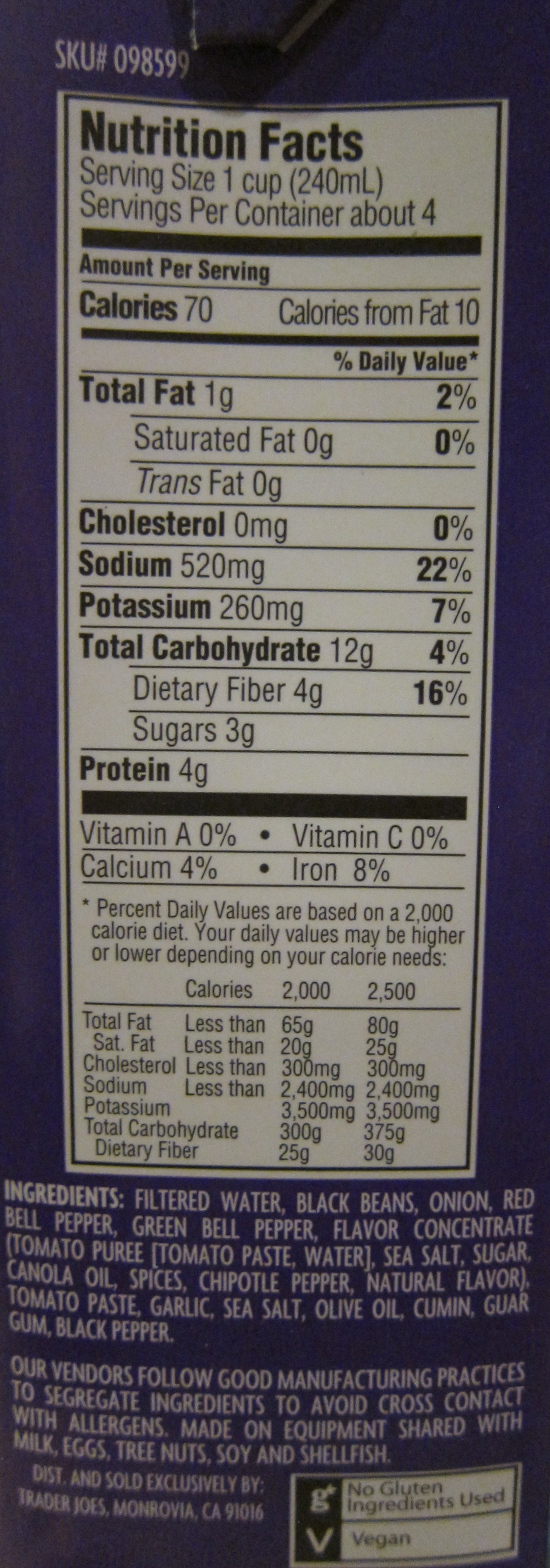Here is a cleaned-up and detailed caption for the image:

---

This image showcases the side panel of a food item, specifically a carton of soup from Trader Joe's with a dark purple packaging. The SKU number is 0-9-8-5-9-9. The panel prominently features the nutrition facts and ingredient list. The serving size is one cup (240 milliliters), with approximately four servings per container. Each serving contains 70 calories, 10 of which are from fat. 

Nutritional breakdown per serving:
- Total Fat: 1 gram (2% DV)
- Saturated Fat: 0 grams (0% DV)
- Trans Fat: 0 grams
- Cholesterol: 0 milligrams (0% DV)
- Sodium: 520 milligrams (22% DV)
- Potassium: 260 milligrams (7% DV)
- Total Carbohydrate: 12 grams (4% DV)
- Dietary Fiber: 4 grams (16% DV)
- Sugars: 3 grams
- Protein: 4 grams
- Vitamin A: 0%
- Vitamin C: 0%
- Calcium: 4%
- Iron: 8%

The % Daily Values are based on a 2,000 calorie diet. Your daily values may vary based on your caloric needs.

**Ingredients:** Filtered water, black beans, onion, red bell pepper, green bell pepper, flavor concentrate (tomato puree made from tomato paste and water), sea salt, sugar, canola oil, spices, chipotle pepper, natural flavor, tomato paste, garlic, sea salt, olive oil, cumin, oregano, black pepper.

It also states that their vendors follow good manufacturing practices to prevent cross-contact with allergens. The soup is made on equipment that is shared with milk, eggs, tree nuts, soy, and shellfish. The product is distributed and sold exclusively by Trader Joe’s.

---